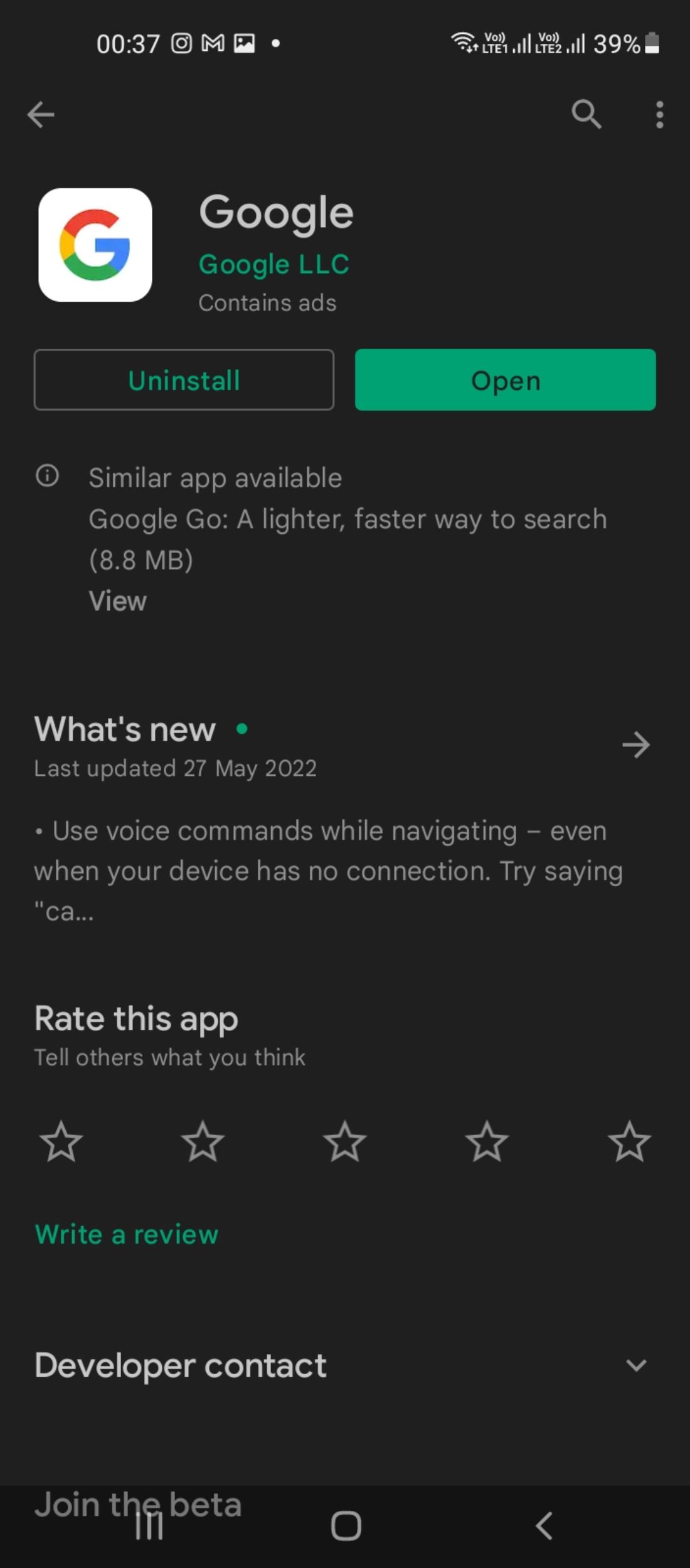This is a detailed screenshot from a smartphone display with a black background. At the top of the screen, it shows the time "00:37," flanked by phone status icons for Instagram, Gmail, Wi-Fi signal, and network coverage, with the battery indicator showing 39% charge. Just below this top bar, there is a navigational and functional toolbar that includes a left-pointing white arrow, a magnifying glass icon for search, and three vertical dots representing additional options.

Below this toolbar, there is a white square icon with the Google logo on it. To the right of this icon, the text reads "Google" with "Google LLC" listed beneath it. This section also includes the notations "Contains ads," alongside options to "Uninstall" and "Open" the app. The "Open" button has been selected.

Further down, a prompt indicates the availability of a similar app named "Google Go," described as a lighter and faster way to search, with a download size of 8.8 MB. It also offers a "View" button to explore this alternative.

The section titled "What's new?" reveals that the app was last updated on 27 May 2022 and introduces a feature that allows the use of voice commands while navigating, even when the device is offline. The example given is to try saying "CA...".

Below this update, there is an option to "Rate this app" with five star icons available for rating, alongside a prompt to "Write a review." Additionally, there are options for "Developer contact" and a prompt to "Join the beta."

At the bottom of the screenshot, three navigation icons are visible: three vertical lines, a white square, and a white arrow pointing to the left. The overall screenshot is vertically oriented, being taller than it is wide.